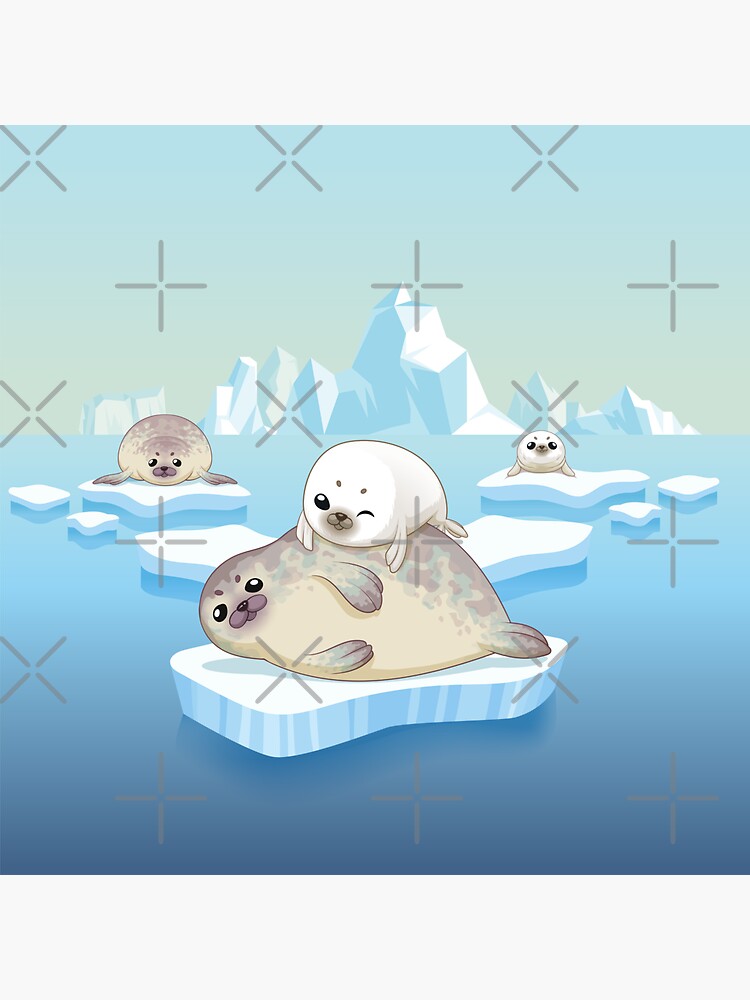The image portrays a whimsical cartoon scene featuring seals lounging on floating icebergs amidst a blue-green body of water under a gradating sky transitioning from a pale blue to a yellow hue. In the foreground, a large gray seal, tinged with a pinkish hue, is reclined on its side atop a chunk of ice, looking towards the viewer. Resting playfully on the larger seal's back is an adorable white baby seal, winking at the camera. Surrounding this captivating duo, the background reveals additional icebergs upon which other seals reside. To the left, another adult seal with a similar grayish-pink hue lies on its stomach, facing the viewer, while to the right, a white baby seal mirrors this position. The tranquil scene is set against a backdrop of towering glaciers that hint at pieces breaking off and forming the smaller icebergs. Adding a touch of graphic charm, the sky above is dotted with alternating rows of X's and plus signs, enhancing the whimsical nature of the illustration.